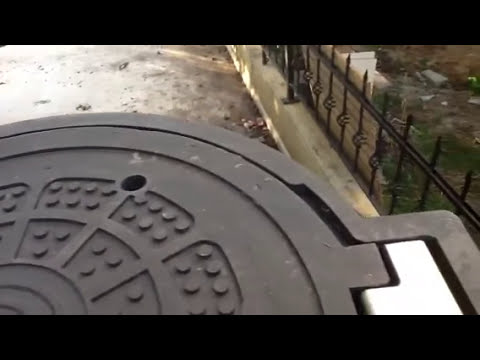In this outdoor photograph taken near a park, the foreground prominently features a partial view of a round, black metallic manhole cover adorned with indented circles. The ground around the manhole appears dark from dirt and soil. To the right, a black wrought iron fence with sharp, spiky posts stands roughly two feet high, marking the boundary of the walkway. In the background, a glistening wet concrete path reflects the sunlight, leading to a green and brown patch of grass. A headstone is also visible near the fence, adding a solemn touch to the scene. The image is bordered by two horizontal black strips on the top and bottom, framing the composition.